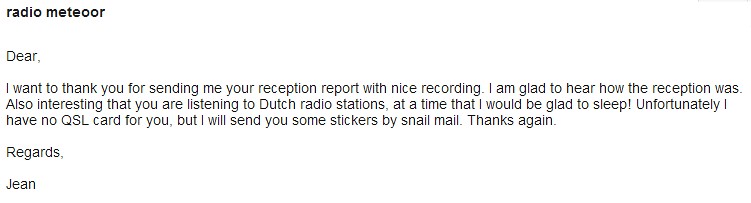This image features a straightforward screenshot of an email displayed against a white background with black text. Centered prominently, the email begins with the bold lowercase title "radio meteor" followed by "Dear" in standard text. The body of the message appreciates the recipient's reception report and expresses interest in their engagement with Dutch radio stations, even while the sender would prefer to sleep. It continues with an apology for not having a QSL card but promises to send stickers via snail mail. The email concludes with "Thanks again" and "Regards," followed by the signature "Jean." The clean, minimalist format emphasizes the clear communication and polite tone of the correspondence.